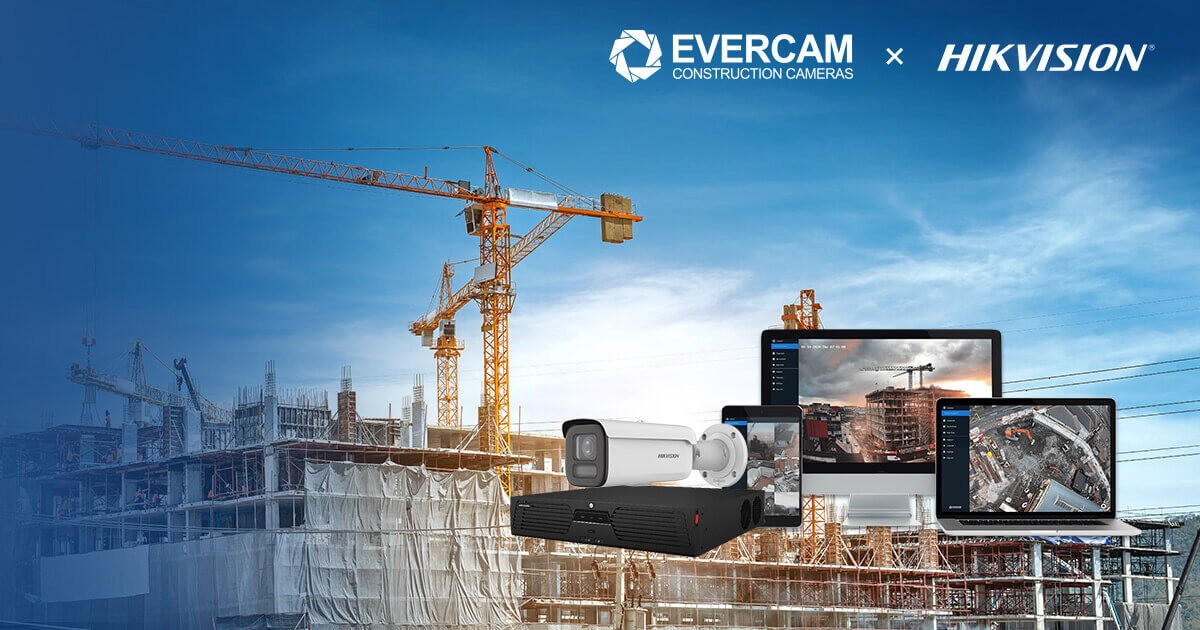The image is an advertisement prominently featuring the text "EverCam, construction cameras" in bold white letters in the upper middle. To the right of this, there is a multiplication sign (X), followed by "HikVision" in a trendy italicized font. Dominating the background, a large industrial construction site is depicted, showcasing several cranes – a smaller one in the back, a large one in the front, and a medium one in the middle – all working together to build a massive multi-story structure. Visible scaffolding and intricate metalwork frame the burgeoning building. The sky is a clear blue adorned with wispy white clouds. In the bottom right corner of the image, multiple devices are displayed, including a white security camera with a gray front, which is positioned beside various tablets, monitors, and a laptop, seemingly used for tracking construction progress. Below the camera, there is a black device resembling an old-time VCR.